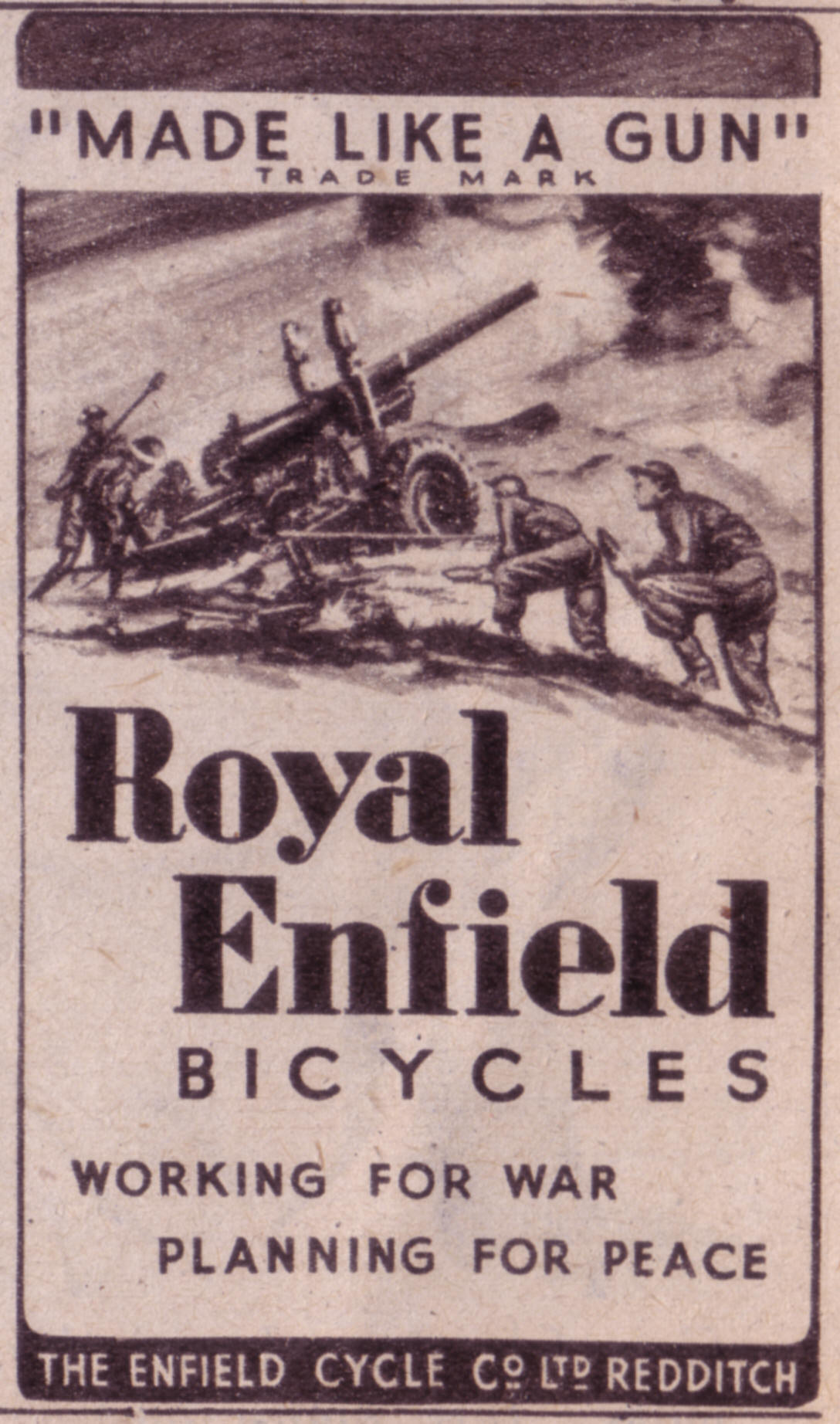The image appears to be a vintage black-and-white tin sign, possibly originating from an old newspaper advertisement. It features a detailed battlefield scene with three to four soldiers operating a military cannon on wheels. Smoke, and perhaps a flame, emanate from the cannon as it fires into the distance. The soldiers are depicted in various crouched positions, possibly trying to evade return fire.

The sign has several textual elements. At the top, a white banner displays the quote, "Made like a gun," followed by a trademark symbol. Below this banner, the words "Royal Enfield" are prominently printed in heavy black font, with "Bicycles" in smaller print beneath. Further down, in even smaller text, the phrase "Working for war, planning for peace" is visible. Finally, at the bottom of the sign is a black banner carrying the text "The Enfield Cycle Co. Ltd., Redditch." This detailed composition provides a snapshot of the historical branding and marketing techniques of the era.